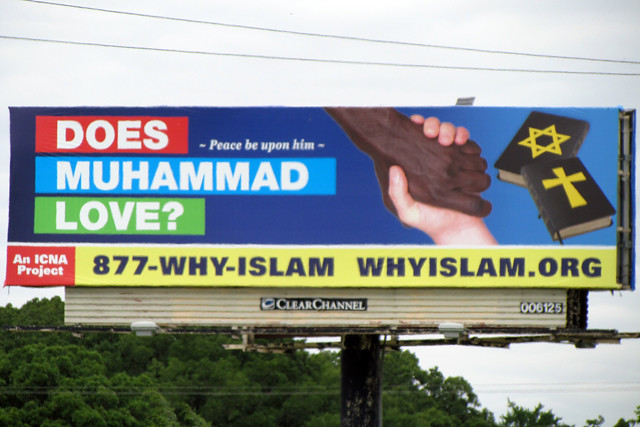This captivating image showcases a towering billboard mounted on a thick, sturdy black metal pole, standing prominently against a backdrop of treetops. The sky above is a soft, light blue, partially obscured by an expanse of fluffy white clouds, indicating a somewhat overcast day. The billboard itself is striking, featuring a poignant image of a black man’s hand clasping a white man’s hand in a handshake, symbolizing unity and peace. Bold text on the billboard poses the thought-provoking question, "Peace be upon him. Does Muhammad love?" followed by a contact reference to 877-Y-Islam.org. To the right of the text, there are images of two religious books, one adorned with a cross and the other with the Star of David, highlighting a theme of interfaith dialogue and respect.